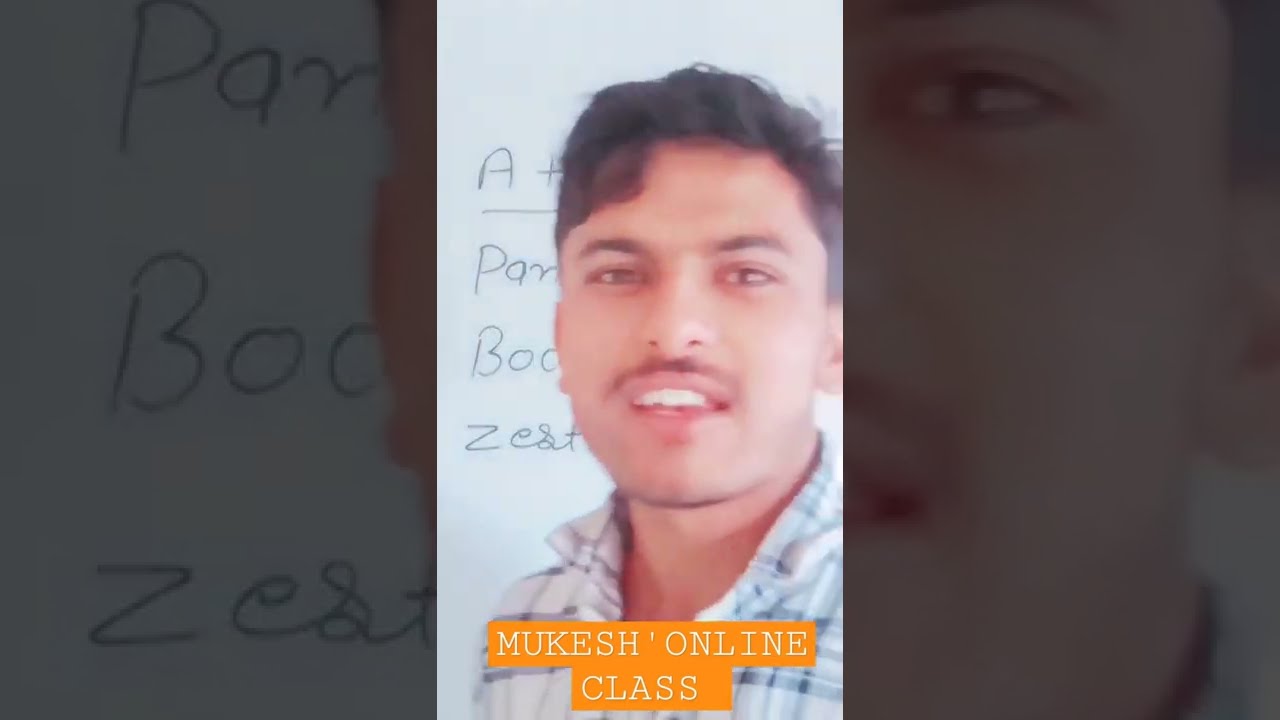This image is a screenshot captured from a video, likely a social media clip or an online class, given the smartphone aspect ratio. The focus is on a young man, possibly in his late 20s or early 30s, who appears to have Middle Eastern features. He has short, dark brown hair and sports a thin mustache with a bit of facial hair on his chin. He's smiling slightly, exposing his white teeth, giving the impression he might be mid-sentence. He is dressed in a white button-up shirt with a blue plaid pattern.

The background features a whiteboard filled with various words, though they are mostly obscured or difficult to fully discern. Notable visible text includes a capital 'A', 'PA', 'B-O-O-Z-E-S-T', and 'Pam', suggesting some kind of instructional or note-taking context. Prominently, there is text at the bottom of the image on an orange background, which reads in white, block letters: "Mukesh's Online Class." The setup implies that the man might be an instructor or presenter, possibly conducting a virtual lesson.

Additionally, the image includes two small black and white rectangles on either side of the man, which appear to be close-ups of parts of the whiteboard or his face, though they are blackened out. Overall, the context points to an educator engaged in a digital teaching session, with details of the whiteboard content partially visible but not entirely clear.